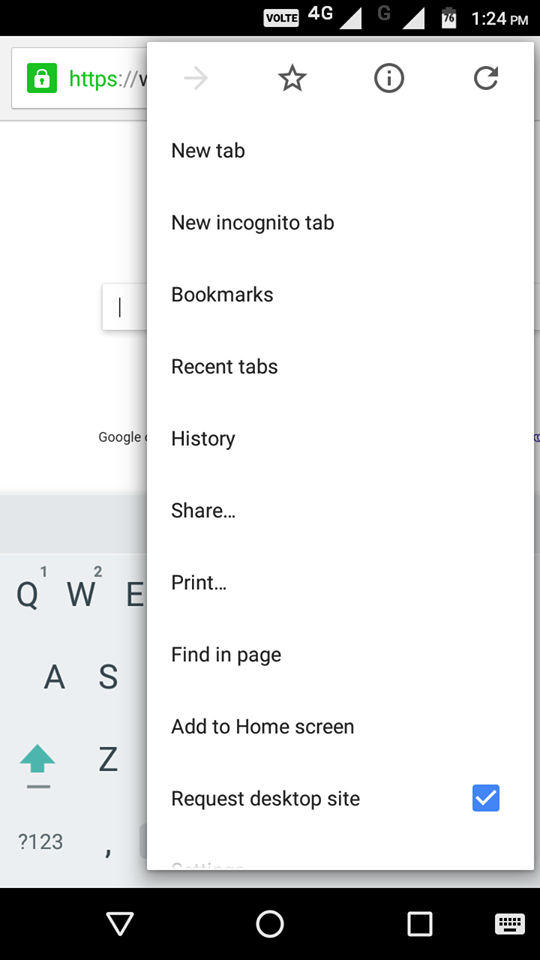**Detailed Screenshot Description:**

This image is a detailed screenshot from a smartphone display, encapsulated with black borders – approximately half an inch at the top and about an inch at the bottom. Positioned along the top edge of the screenshot, there's a centered white rectangle within the black border that displays "V-O-L-T-E" in black text. Adjacent to this, on the right, are indicators showing "4G," a fully filled Wi-Fi icon, another full Wi-Fi bar, and a battery icon displaying "76%," followed by the current time, "1:24 p.m."

Overlapping the right side of the screen, a white rectangular section extends about two-thirds down from the top. This rectangle features a gray border running along its left, right, top, and bottom edges. Within this segment, there's a partially visible search tab showcasing a green square with a white lock icon, denoting "HTTPS://". Continuing below this search tab is a white background containing the word "Google" in large black letters situated towards the bottom of this white section.

Beneath the white rectangle, a portion of the on-screen keyboard is visible. The top row displays the characters "Q-W-E-R-T-Y," and part of the second row shows "A-S-D" with a blue arrow next to the "Z." There's a "question mark," along with the keys "1-2-3" and a comma in the keyboard's popup tab.

Further up on the right-hand side of the white rectangle, various function icons can be seen: a grey arrow pointing right, a black star, a small black circle containing an "i," and a refresh button. Below these function icons, there are tab options for the user to click on, with the bottom-most option, "Request Desktop Site," highlighted with a blue square and a white checkmark.

Lastly, the bottom black border of the screenshot includes several icons: an upside-down triangle, a circle, and a square – each icon bordered in white with a black interior. There is also a calendar icon depicted as white with black dots. These are likely part of the smartphone's navigation and menu options.